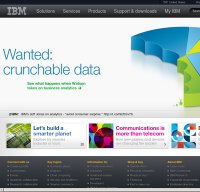In this blurry and grainy screenshot, a black header at the top prominently displays the IBM logo in block letters. To the right of the logo, there are grey words that are difficult to make out, except for the word "Solutions" and a button labeled "Products." Below the header, on a light grey background, the blue text reads "Wanted: Crunchable Data." Underneath this, there is some green text that is illegible, accompanied by a right-pointing arrow.

On the right side of the image, there is a digital graphic resembling a pie chart in blue, green, and yellow hues, with several bites taken out of its left side. Beneath this, there is a square image with an abstract design featuring blues, greens, blacks, and greys. Further to the right, text reads "Let's Build a Smarter," followed by an indistinct word. Adjacent to this text, there's another abstract graphic in pink, blue, yellow, and purple tones, with the pink text "Communications In" partially visible.